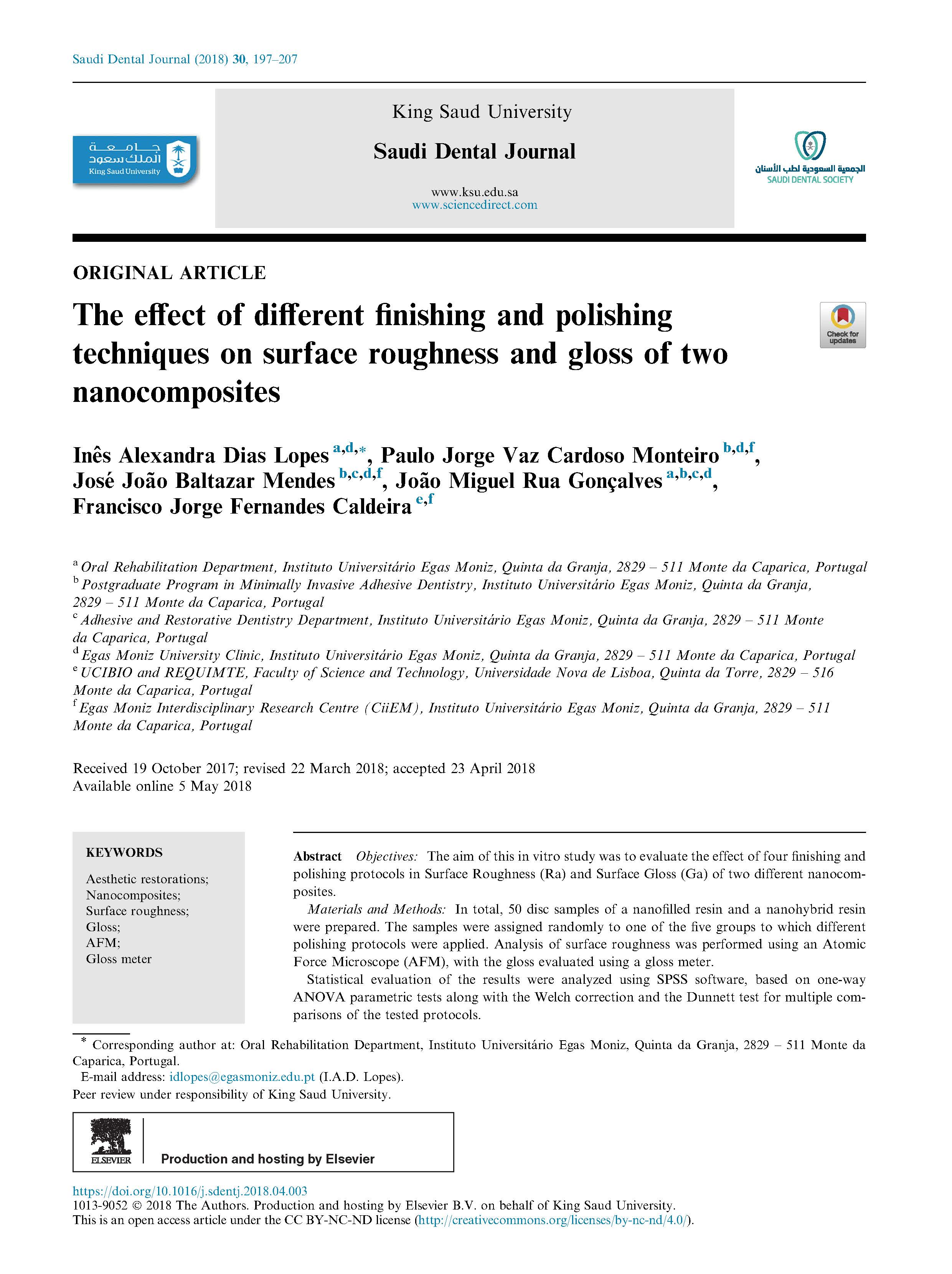This photo displays the front page of an issue from the Saudi Dental Journal, specifically featuring an article from King-Sumpton University. The title of the research article, highlighted in bold, reads, "The Effect of Different Finishing and Polishing Techniques on Surface Roughness and Gloss of Two Nanocomposites." Below the title, a list of five contributing authors is presented.

The abstract of the article follows, written in a script-like font and a light color, making it somewhat difficult to read. This section encompasses one or two brief paragraphs summarizing the study.

Further down the page, the submission and publication timeline is detailed, noting the dates as follows: received on October 19, 2017, revised on March 22, 2018, accepted on April 23, 2018, and made available online in May 2018 (specific date is unclear, possibly May 14 or May 18).

A small blue box labeled "Keywords" is positioned below this section, listing pertinent terms related to the article for indexing purposes. To the right of this box, another section contains a couple of paragraphs, which likely provide additional context or a brief introduction related to the research.

At the bottom of the page, catalog and website information is provided, presumably to guide readers to further resources or related articles on the journal's platform.